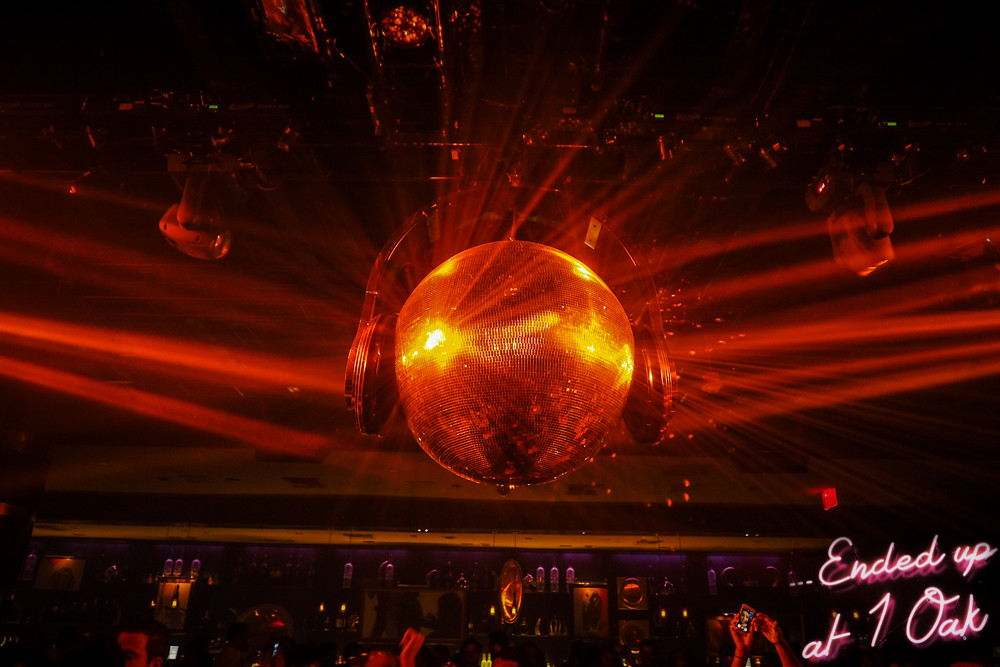In this vibrant and creative full-color photograph taken inside a buzzing nightclub, a colossal disco ball adorned with headphones commands the center stage. Bathed in golden light that it deftly refracts across the room, the disco ball exudes a mesmerizing glow with flickers of red and yellow hues, setting a lively and uplifting atmosphere. High above the crowd, the disco ball's reflections intertwine with other ceiling lights, creating a dynamic interplay of illumination. Below, shadows and silhouettes of dancers are faintly visible, their hands raised in jubilation, contributing to the spirited ambiance. This promotional piece for "1 OAK" is subtly marked in the lower right corner with the phrase "ended up at 1 OAK" in a chic pink and white cursive font, inviting onlookers to join in the revelry at this pulsating venue.